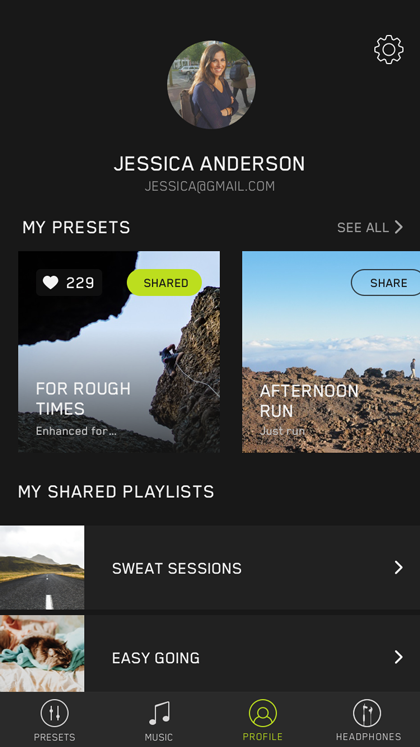This is a detailed screenshot of Jessica Anderson's profile on a music app. The top of the profile features a vibrant picture of Jessica, likely taken outdoors. She has long, dirty blonde hair and stands with her arms crossed, exuding a happy and confident demeanor. Her gaze is directed at the viewer, although her body is slightly angled to the side. In the top right corner of the profile image, there's a gear icon, presumably for accessing settings.

Below her name, "Jessica Anderson," there's a link to her personal website, JessicaAnderson.com. Following this, a section titled "My Presets" is displayed, showcasing a music playlist named "Reptimes." This playlist is marked as shared, evidenced by a green "shared" button in the top right corner of the playlist section, and it has garnered 229 likes, indicated by the heart icon on the top left.

Underneath the "Reptimes" playlist, there are additional sections labeled "Afternoon Run," "Sweat Sessions," and "Easygoing." Each of these presumably represents different music playlists or categories curated by Jessica.

At the bottom of the screenshot, there are several navigation tabs, with the "profile" tab highlighted in green, indicating that this is the currently selected section.